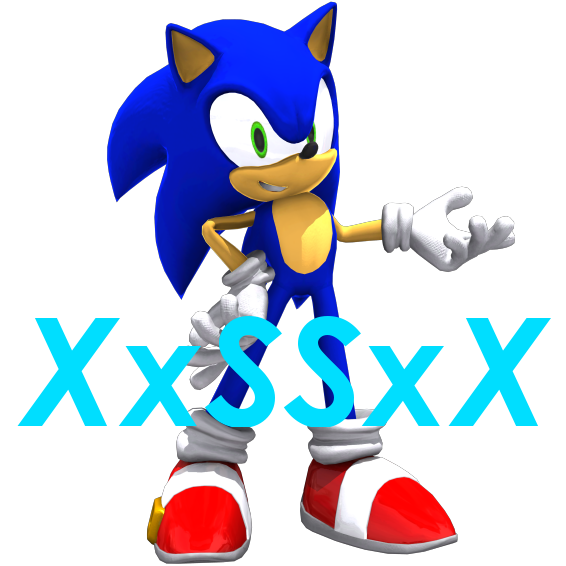This image features a detailed digital depiction of Sonic the Hedgehog, the iconic video game character, standing confidently. Sonic's body is primarily bright blue, with a large head, pointed ears, and green eyes with black pupils. He has a distinct muzzle and mouth that are yellow, while his chest and arms appear in a peachy tan hue. Sonic's nose is black, and partial white teeth peek out from his yellow face.

Sonic is wearing his signature large white gloves, which accentuate his expressive hands—one resting on his hip and the other extended outward. His legs are skinny and blue, leading down to his characteristic red and white running shoes, which feature a white stripe and gold buckles on the sides. Completing his footwear are white scrunchie socks.

Across the image are broken up blue letters "XXSSXX," serving as a visible watermark. Though part of the watermark is difficult to discern, it is clear against Sonic’s vivid colors and some of the lighter parts of the background. The overall composition blends Sonic's classic features with additional textual elements to create a vibrant and detailed portrait.